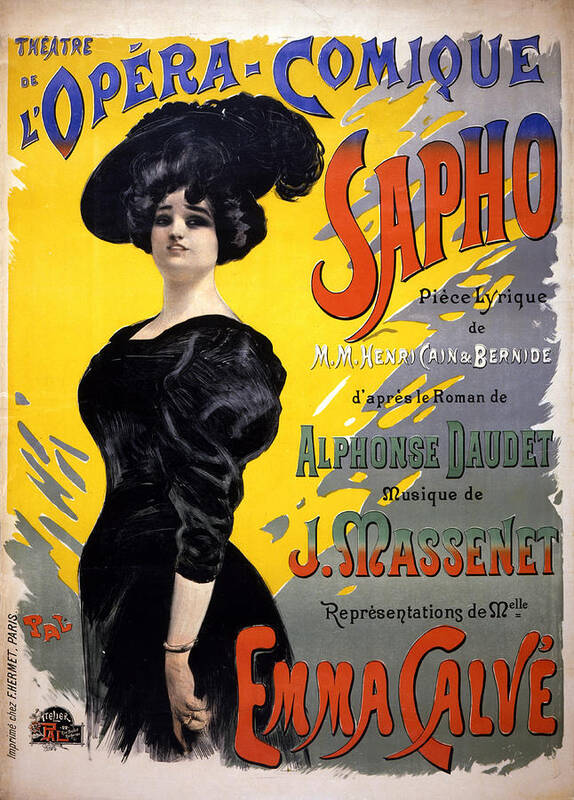This image is the cover or a poster advertising an older French opera titled "Théâtre de l'Opéra Comique: Sappho." The poster features a detailed drawing of a stout woman with dark black hair, adorned with a large, frilly black hat. She is elegantly dressed in a black dress with puffed shoulders and sleeves, complemented by a bracelet on her left wrist and a possible wedding band. The background of the poster is predominantly yellow with some gray accents. 

The text is in French and provides detailed information about the opera, identifying it as a piece lyrique by M.M. Henry Cain and Bernard, based on the novel by Alphonse Daudet. The music is composed by J. Massenet. The poster also highlights the performances by the renowned singer Emma Calvé. Overall, this color poster is a meticulously drawn advertisement that showcases the elegance and classic style of the period in which it was created.